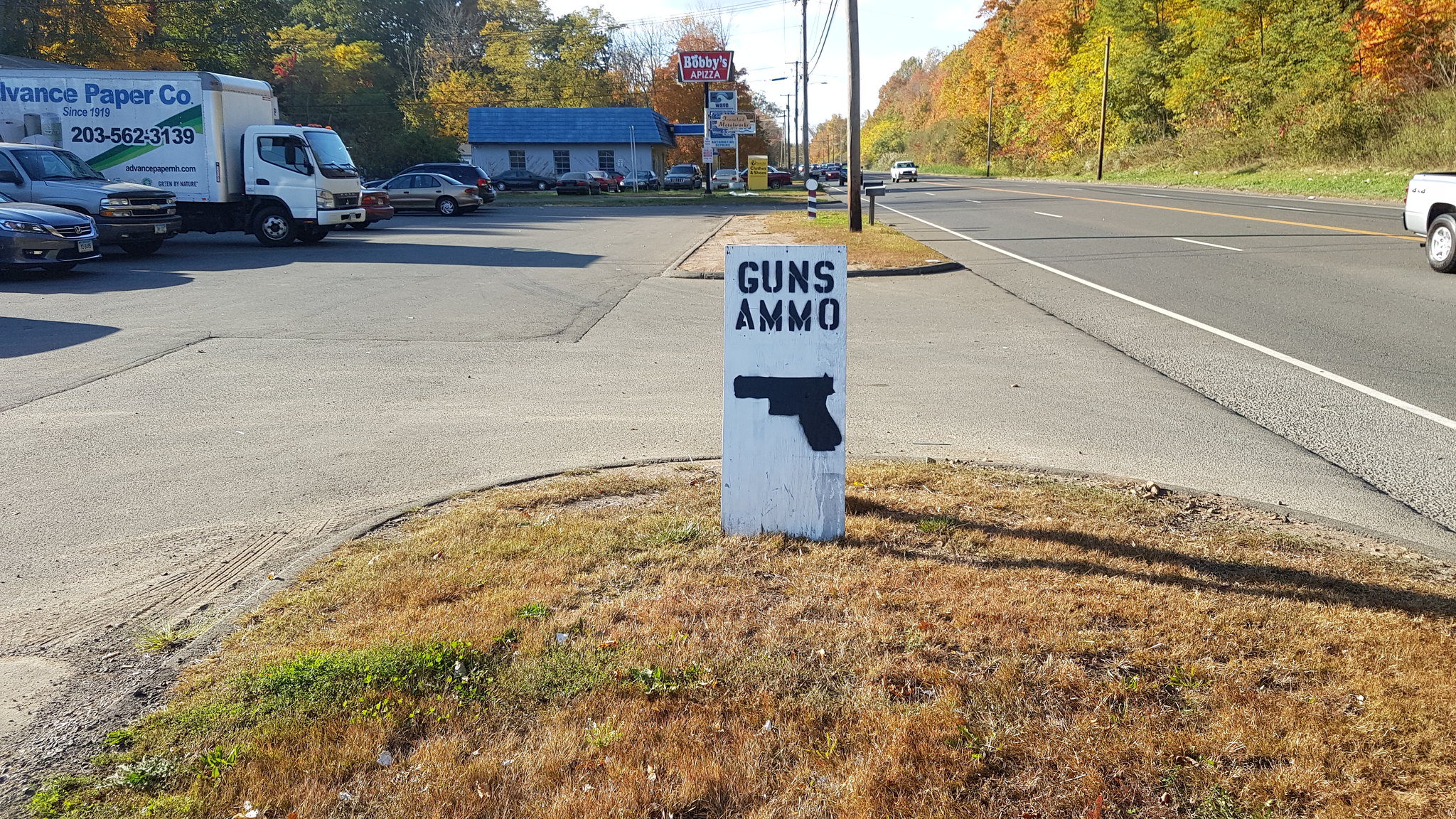The image is a daytime outdoor scene, approximately one and a half times wider than it is tall, captured during the fall under a partly cloudy sky. The primary focus is a four-lane road with southbound traffic, located to the right of the frame, lined by trees transitioning into autumn hues of green, red, orange, and yellow. To the left of the road is a strip mall with a variety of businesses, most notably featuring a hard-to-read red sign possibly indicating "Bibby's Pizza." Other businesses are present, set in a light blue building with a blue roof.

In the middle ground, a predominantly dead grassy area occupies much of the image. A prominent white vertical sign stands within this grass, displaying "GUNS AMMO" in black letters and featuring a black handgun symbol that doubles as a directional arrow pointing left. This sign directs to a parking lot on the left side of the image, filled with several parked cars, including a noticeable white truck with an attached large storage area. In the distance, the tree line displays a mix of fall colors similar to those along the road. Further left in the background, additional businesses can be noted, including one with a visible portion of a sign reading "Vance Paper Company" with a phone number.